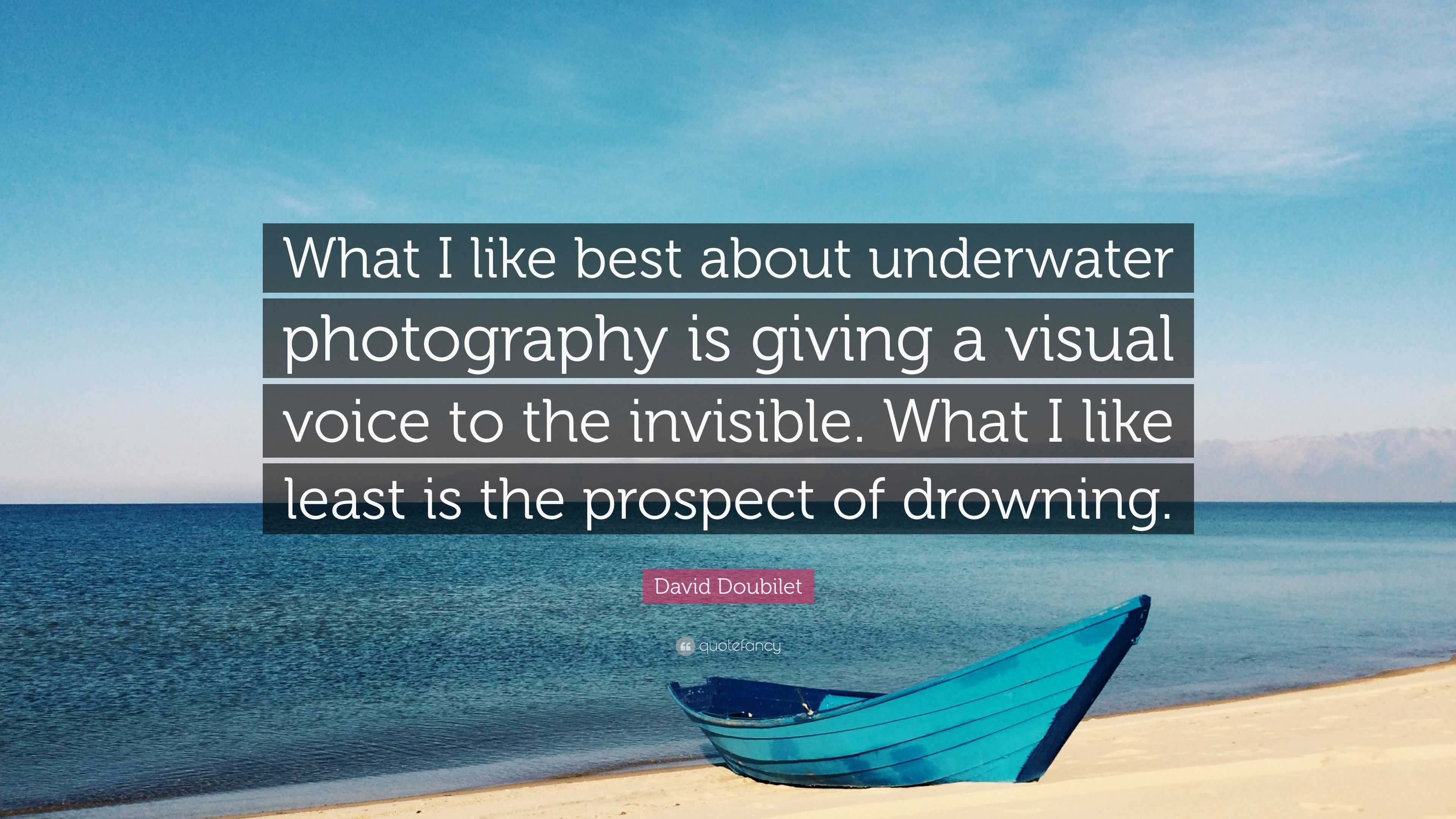The image features a serene beach scene with a bright blue, perhaps teal, rowboat resting on the tan sand where it meets the calm ocean water. In the distance, a small mountain can be seen. The sky above is largely clear with light blue hues and a few wispy clouds. Central to the image is a prominent quote superimposed in white text inside semi-transparent black rectangles, with each line of the quote in its own rectangle. The quote reads: "What I like best about underwater photography is giving a visual voice to the invisible. What I like least is the prospect of drowning." Beneath this quote, in a pinkish-purple rectangle, the name "David Doubilet" is displayed, alongside an unreadable watermark. The overall effect of the image is somewhat illustrative rather than photographic.